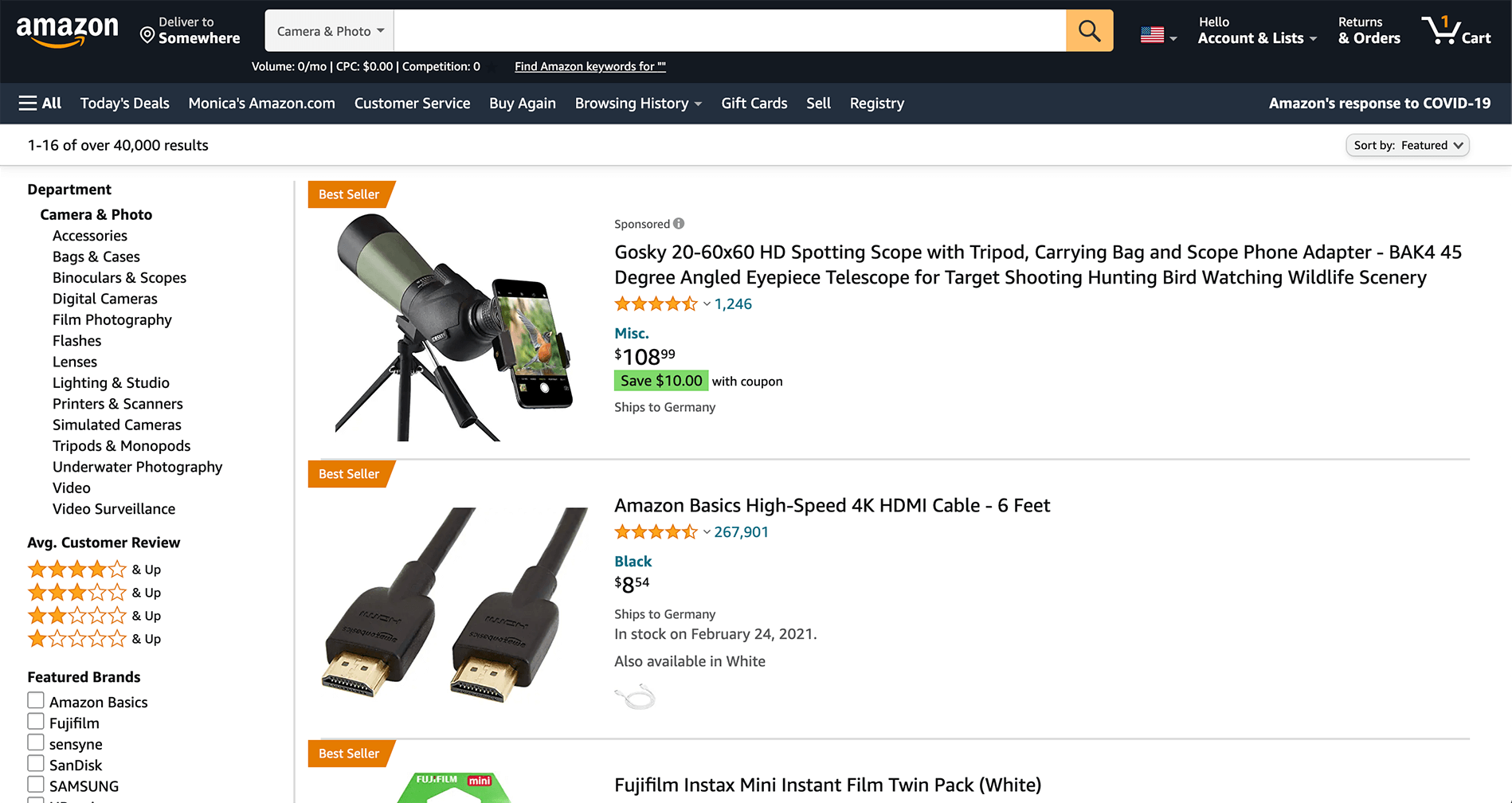This image is a detailed screenshot of an Amazon webpage. 

At the top, the iconic Amazon logo is prominently displayed. To its right, there's an option labeled "Deliver to" allowing users to select their location. Following that is a search bar with "Camera & Photo" pre-selected from a dropdown menu on the left side. Beside the search bar is a yellow search button. Adjacent to the search bar is the United States flag symbol which allows for country selection.

Next to the country selector, there's a greeting that says "Hello, Account & Lists" which is a dropdown menu, followed by a "Returns & Orders" button. There is also a shopping cart icon indicating that there is one item currently in the cart.

Below this top navigation section, there is a menu with a "See All" option. On the right-hand side of the page, in bold white text, is a message about “Amazon's response to COVID-19”.

The main content of the page shows two search results. The first result is for a “Gosky HD Spotting Scope with Tripod, Carrying Bag, and Scope Phone Adapter,” priced at $108.99. This item is marked as one of their best sellers and offers a coupon to save $10. The second result is for an "AmazonBasics HDMI Cable - 6 Feet", priced at $8.54. This item is black in color and also tagged as one of their best sellers.

On the left-hand side of the page is a detailed sidebar. It starts with a departmental list where "Camera & Photo" is pre-selected. Underneath, there is an "Average Customer Review" section which allows users to sort products based on customer reviews. Further down, there is a "Featured Brands" section where users can filter products by brand.